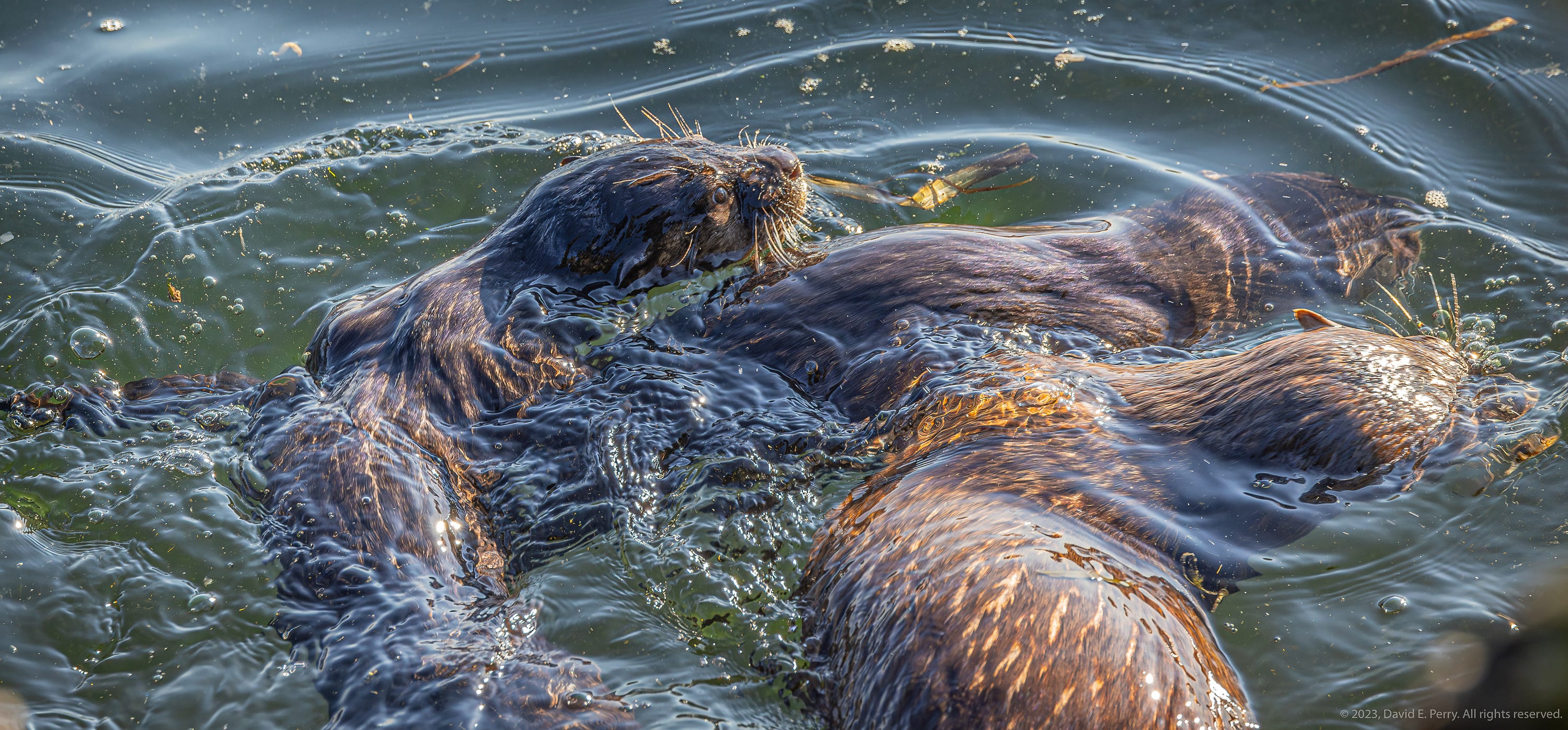This image is a well-lit, realistic outdoor photograph taken in a horizontal rectangular format that is wide but not very tall. It captures a serene nature scene featuring a body of dark, almost muddy, water with subtle ripples. In the water, there are three to four brown-furred animals—identified as either otters, beavers, or sea lions. These animals are swimming close together, with their heads and some parts of their bodies visible above the water. Their fur reflects white light, likely from the Sun, adding a glistening effect to the scene.

In the image, one animal is prominently displayed in the upper left-hand corner, showing its head with visible whiskers and dark, blackish-brown fur. Another one is slightly below it, facing to the right, with a clear view of the top of its head and whiskers. The third animal, located toward the middle, has only its back visible, and another to the right of it shows most of its back and some of its head peeking out of the water, looking away from the camera.

There is a barely noticeable small white font in the bottom right corner that reads "2023 David E. Perry All Rights Reserved." The overall peaceful atmosphere is further enhanced by the minimal ripples made by the swimming animals, suggesting they are enjoying their time in the water.